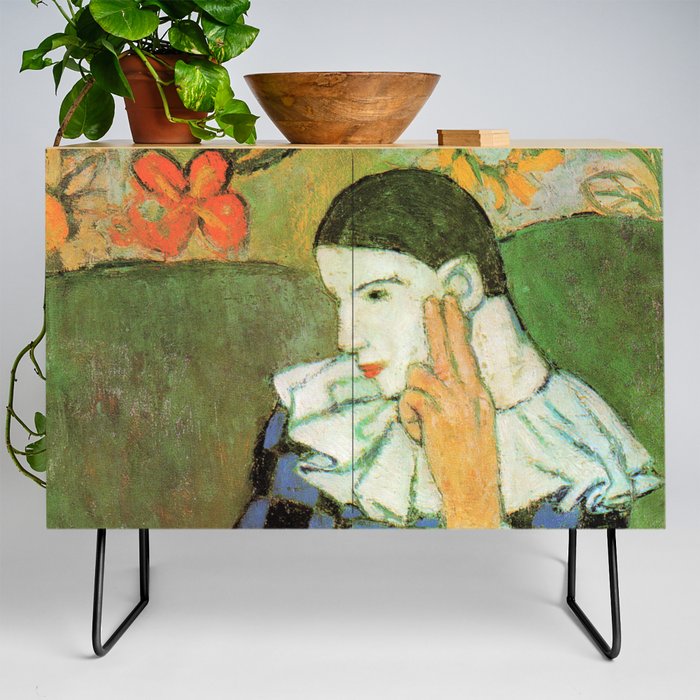The image depicts a unique piece of functional art furniture, possibly an end table or credenza, adorned with a digitally enhanced representation of Pablo Picasso's early 20th-century painting "Harlequin Resting on His Elbow." This striking piece features the iconic portrait of a young harlequin with pale white skin, bright red lips, and slicked, flat black-green hair. The harlequin's left hand, in natural flesh tones, gently touches his ear with two fingers extended while the others are folded inward. He wears a white ruffled collar over a dark blue and black patchwork outfit, set against a predominantly green background accented with gray, brown, and black hues, along with a stylistic red flower.

On top of the credenza, a medium-colored wooden bowl and a stack of wooden coasters contribute to the decor. A terracotta pot, with a green ivy plant cascading over its edges, adds a touch of nature. The overall scene combines classical art with contemporary home decor, offering a vivid and detailed glimpse into the harmonious blend of functionality and aesthetic appeal.